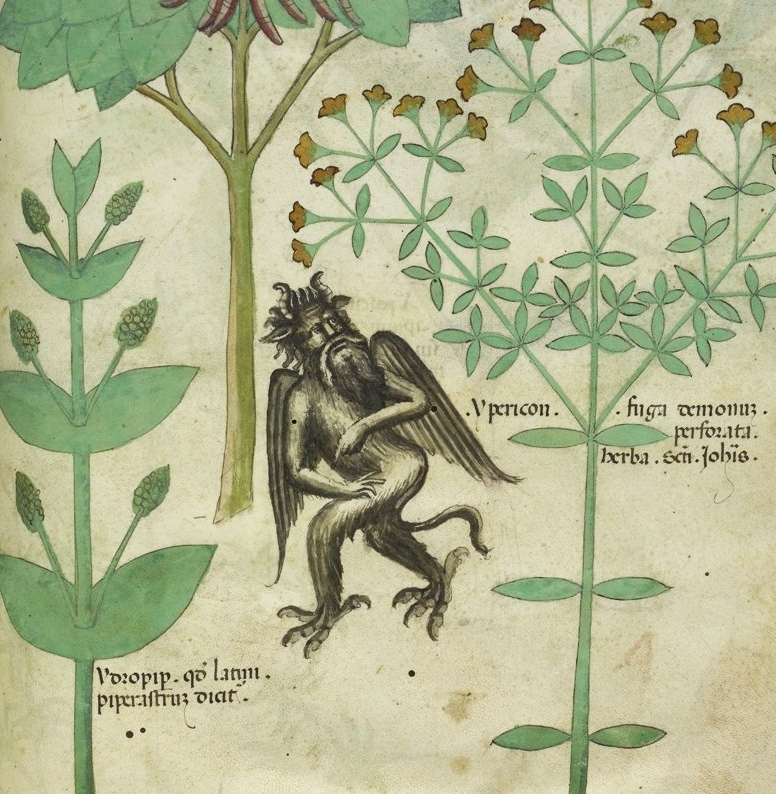The image is a print or poster set against a grayish background, featuring lush green plants on both the left and right sides. The plant on the left side has big leaves attached to thin stem branches terminating in leaf pods adorned with numerous circles, possibly buds. The right side showcases a very tall plant that branches out, boasting yellow-brownish flowers clustered around the upper tips. Just left of this is an olive-green tree with a few branches, barely discernible green leaves, and red, bean-shaped skinny items hanging from it.

Centrally positioned within the foliage is a fantastical creature with a long, furry body that extends down to its bird-like, clawed feet. It stands on two legs, faces slightly sideways, but directs its gaze towards the viewer. The creature has a long beard, dog-like ears sprouting from the sides of its head, and horns that swoop backwards in an S shape. Additional features include wings and a tail, contributing to its angelic yet monstrous appearance. The character’s face appears somewhat human with a widely spread mustache. Overlaying this scene is black text in a non-English language, featuring eccentric lettering such as "LXRBA."